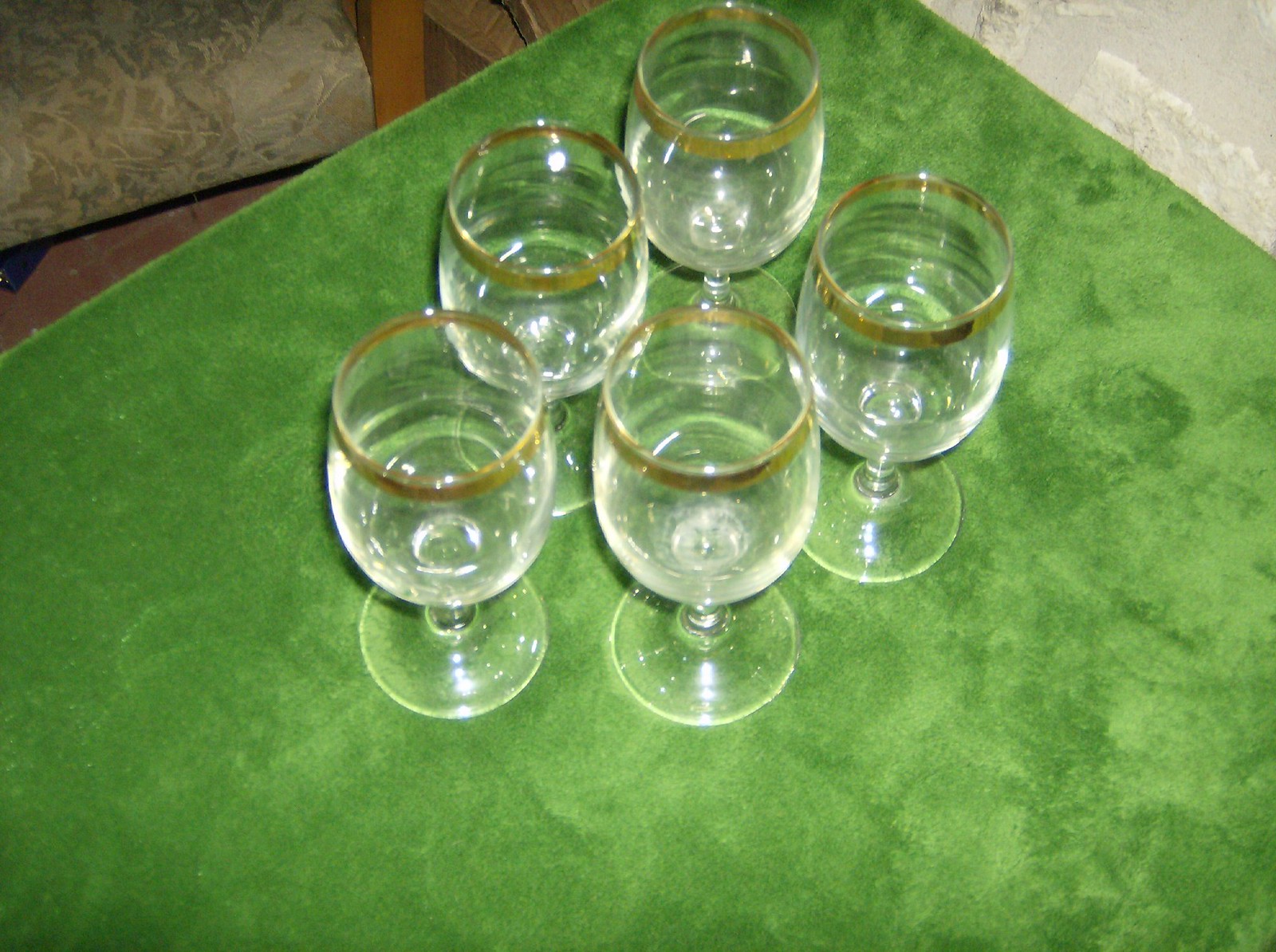In the image, there are five elegant wine glasses arranged closely together on a vibrant velvety green tablecloth, which has a slightly dirty and smeared appearance. The glasses feature a delicate light green and gold rim at the top and long stems ending in a resting glass portion at the bottom. Nearby, on the far left side of the image, there's a light green cushion with a flowery pattern. The setting is up against a white cement block wall. In the background, to the right, there is a beige chair with wooden sides and a dark beige cushion, adding a touch of contrast to the scene. The entire scene has a slightly messy, yet intriguing composition, with the glasses possibly containing water or a clear liquid, reflecting light and appearing shiny.